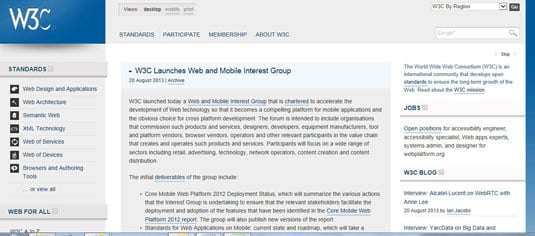The image shows a website with a layout approximately two and a half times wider than it is tall, featuring small text that adds to its visually intricate design. The primary background color is a subtle off-white or gray, providing a neutral canvas for the website's contents.

In the upper left corner is a distinct section with a dark blue background, prominently displaying the W3C logo. The logo consists of a stylized 'W' in a conventional font, followed by a uniquely designed '3' with a squared-off top and diagonal lines forming a triangular shape before transitioning into a rounded bottom. The 'C' in the logo is partially completed, with only the first and bottom thirds visible, giving it a modern and abstract appearance.

Adjacent to the logo on the right, four small buttons are faintly visible, rendered in an extremely small and unreadable font. The upper right corner of the webpage features a dropdown box, although the text within is similarly minuscule and difficult to decipher. Directly below the dropdown box is a search field where users can presumably input queries.

Beneath the top menu, towards the left, there are four additional menu options: "Standards," "Participate," "Membership," and "About W3C." These menu items are part of a broader navigation system aimed at guiding users through the various aspects and offerings of the W3C website.